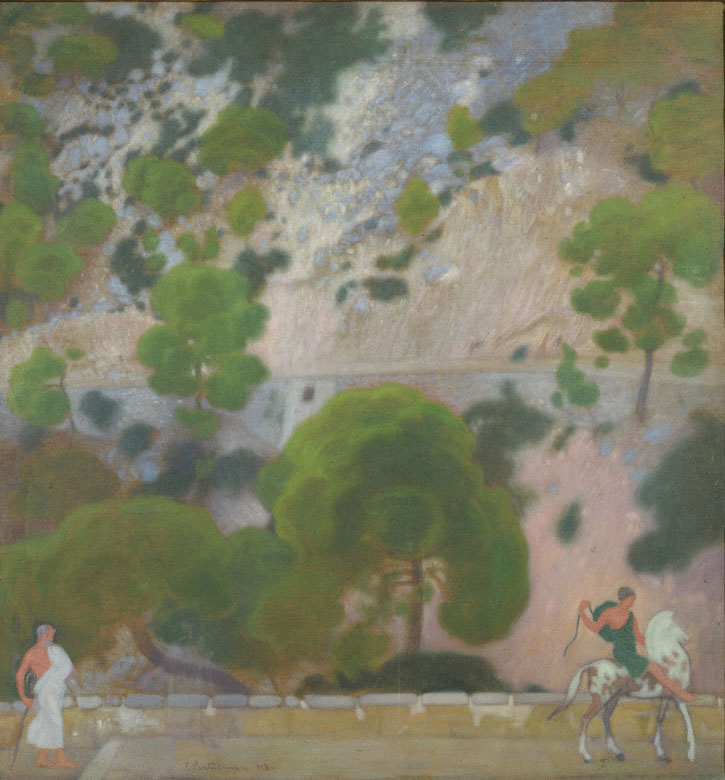The painting depicts a scene reminiscent of Roman times, portrayed through a simplistic watercolor or pastel style with splotchy, muted colors. Central to the image is a white horse with brown or black speckles. Sitting on the horse is a man dressed in a deep green toga, holding something in his hand and having short hair. To the left, another man is seen walking, clad in a white toga and holding a long cane in his right hand. Both figures are set against a backdrop of a rugged landscape, featuring a pathway that is marked by a white picket railing at its edge. Behind the pathway stretches a row of rocks, suggesting the boundary where the road lies. Further back, stems with muted tops depict trees climbing up the side of a granite-colored hill or cliff. These trees are interspersed with bright and dark greens, adding texture to the scene. The background extends upwards, showcasing faint, light-colored areas that convey additional trees scaling the side of a mountain, blending into the overall impression of a serene, ancient landscape.